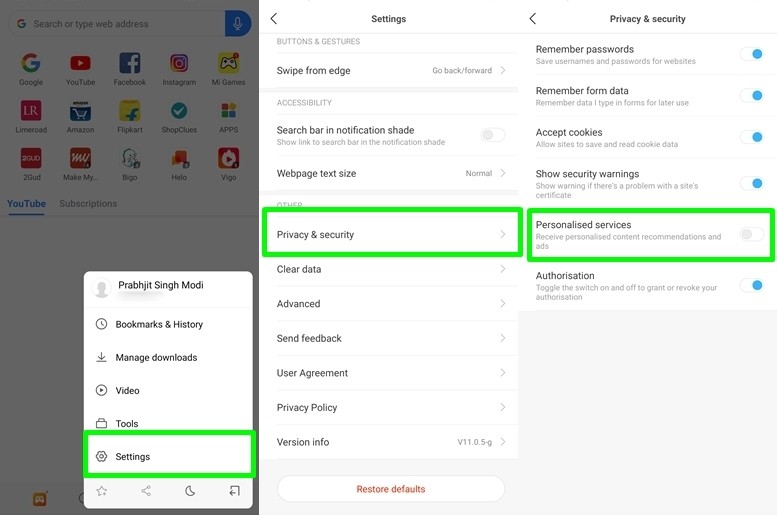A horizontal screenshot, likely from a computer or smart device, is meticulously divided into three vertical sections. The first section, occupying the left third of the image, appears dimmed and displays several familiar icons such as Google, YouTube, Facebook, and Instagram in the background. However, these icons are unclickable, as a white dialog box overlays them in the lower right corner, containing text that reads, "Pravda Deet Singh Modi" along with several options: bookmarks, history, manage downloads, video tools, and settings, the latter highlighted with a green border. Various icons are also arrayed across the bottom of this section.

The central panel is primarily focused on settings. At the top, it shows a settings header followed by options like swipe from edge, accessibility, search bar, notification shade, and web page text size, marked as normal. The category of privacy and security is emphasized with a green-bordered box around it. Notable entries include clear data, advanced settings, feedback, user agreement, privacy policy, version info, and an orange "restore defaults" button at the bottom.

The rightmost section of the image elaborates on privacy and security settings, presented in bold at the top. This section lists several toggled options: remember passwords (activated with a blue circle), remember form data (on with blue), accept cookies (on with blue), show security warnings (on with blue), and personalized services, which is currently off but highlighted by a green rectangular box. The final option, authorization, is toggled on and marked with blue.

Overall, the image presents a detailed glimpse into the settings and privacy configurations of a device or application, indicating various customizable features associated with user data and security.